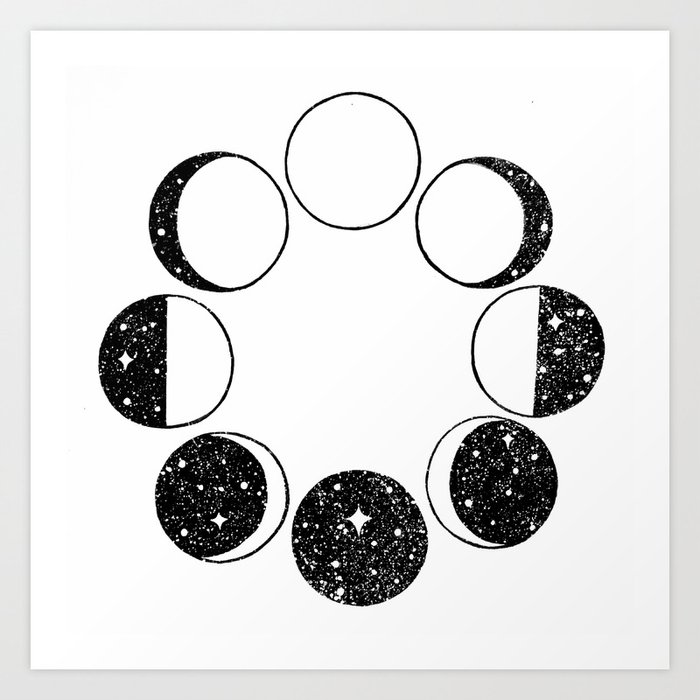The image depicts a detailed, black-and-white illustration of the moon phases arranged in a circular pattern against a solid white background, framed by a light gray border. At the top, the circle positioned at 12 o'clock is outlined in black and completely white. Moving clockwise, the circle at 1 o'clock features a black crescent moon with a three-quarters white circle, adorned with stars in the black portion. The 3 o'clock position shows a perfect half-and-half split of the circle, with the left half black featuring stars and the right half white. Between 4 and 5 o'clock, the circle is three-quarters black with a white crescent moon. At the bottom, the 6 o'clock circle is entirely black, filled with stars. Moving up counterclockwise, the 7 o'clock circle mimics the 4-5 o'clock position but with a crescent moon on the opposite side. The 9 o'clock position again shows a half-and-half composition, but reversed, with the right half white and the left half depicting a starry night sky. Finally, the 10 o'clock circle features a crescent moon made of stars and sky on the left, with a white three-quarters circle on the right. Each stage of the moon phase is meticulously illustrated, transitioning sequentially from a fully white circle at the top to a fully black, star-filled circle at the bottom, resembling an eclipse progression.